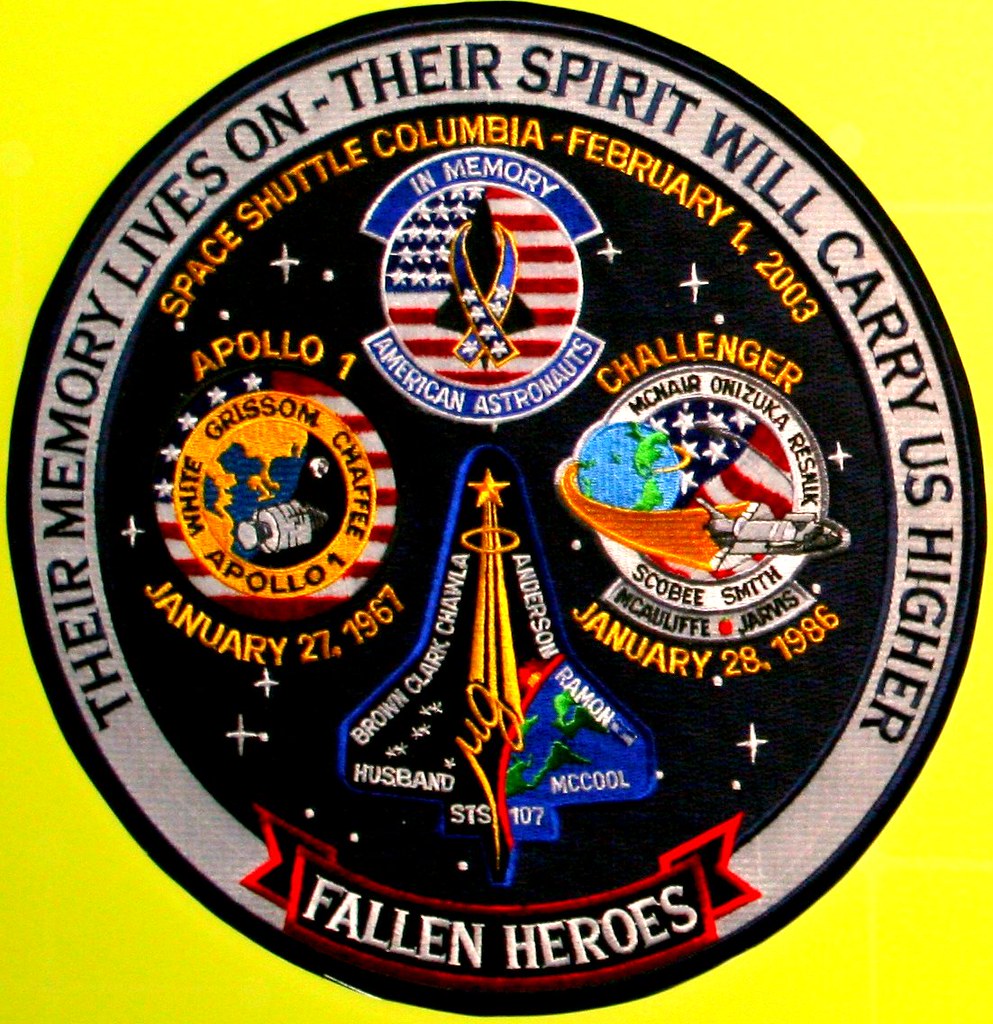This is a detailed NASA commemorative patch honoring fallen astronauts from Apollo 1, Space Shuttle Challenger, and Space Shuttle Columbia missions, set against a yellow background. The circular patch features a black border and a white inner ring with the inscription, "Their memory lives on. Their spirit will carry us higher." Inside, a black circle showcases three distinct mission logos: Apollo 1 (January 27, 1967), Challenger (January 28, 1986), and Columbia (February 1, 2003). The bottom section of the patch displays a red ribbon banner with a black center and white letters reading, "Fallen Heroes." Each mission's logo includes the names of the lost astronauts: Apollo 1 has 'Grissom, White, Chaffee'; Challenger lists 'Smith, McNair, Onizuka, Resnik, Scobee, Jarvis, McAuliffe'; and Columbia features 'Brown, Clark, Chawla, Anderson, Ramon, Husband, McCool.' The centerpiece highlights a space shuttle silhouette outlined in blue with a gold star at the top.